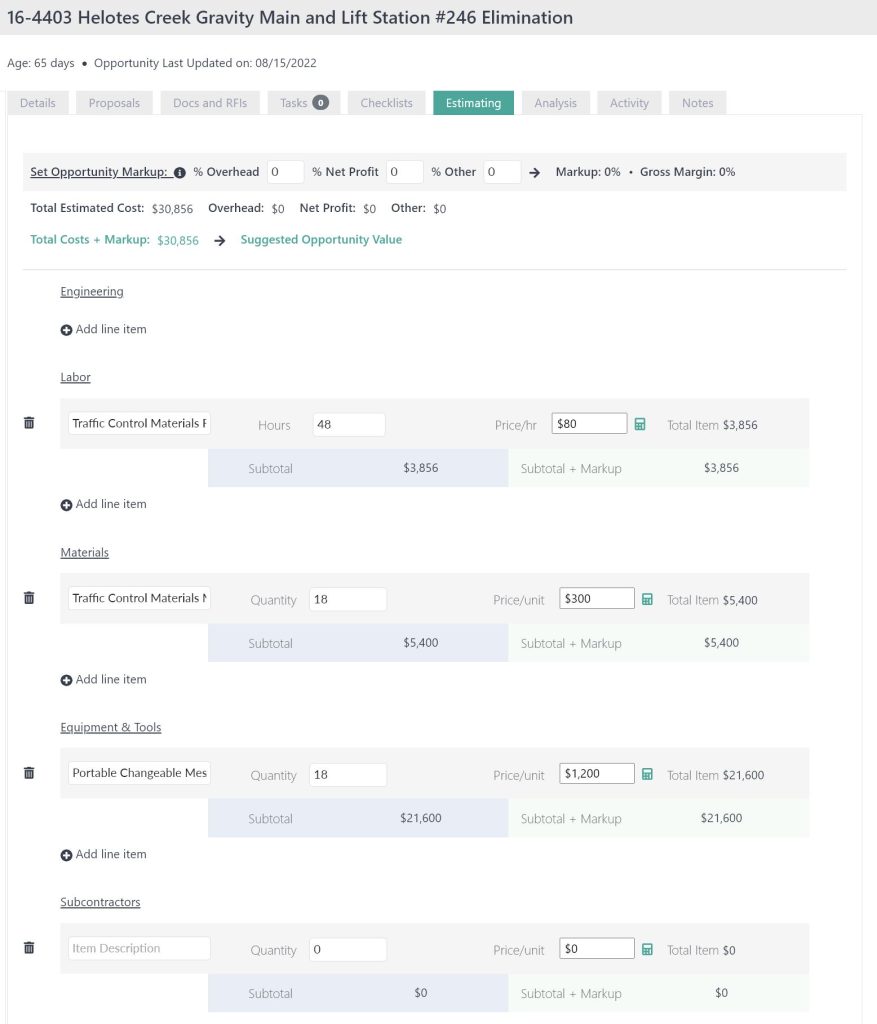This image displays a detailed project banner related to the "16-4403 Pelotis Creek Gravity Main and Lift Station, #246 Elimination". The banner spans horizontally, with a gray background. 

### Top Section:
- **Header:** At the top left, in a white font, the text reads "16-4403 Pelotis Creek Gravity Main and Lift Station, #246 elimination".
- **Sub-heading:** Below, there is a white section indicating "Age: 65 days, Opportunity last updated on 08-15-2022".

### Section Tabs:
- Underneath, several smaller gray tabs with white text include:
  - **Details**
  - **Proposals**
  - **Docs**
  - **RFIs**
  - **Tasks** (indicating a "0" status indicator)
  - **Checklist**
  - **Analysis**
  - **Activity**
  - **Notes**
- **Estimating** stands out in a green banner with white letters.

### Financial Overview:
- Text in black beneath the tabs reads "Set opportunity markup" which has zero values everywhere:
  - **Overhead:** 0%
  - **Net Profit:** 0%
  - **Others:** 0%
- A black arrow precedes further text: "Markup: 0%, Gross Margin: 0%". These zeros appear editable.
- Below, costs are highlighted:
  - **Total Estimated Cost:** $30,856
  - **Overhead:** $0
  - **Net Profit:** $0
  - **Others:** $0
- Written in green: **Total Cost plus Markup:** $30,856
- Followed by another black arrow and green text indicating "Select Suggested Opportunity Value".

### Detailed Breakdown:
- A fine gray line separates the sections, leading to:
  - **Engineering:** (outlined and underlined)
  - **Add Line Item** (with a positive sign)
  - **Labor:** (underlined)
  
**SHOULDERS of Traffic Control Materials include:**
- **Hours:** 48
- **Price per Hour:** $80
- **Total Item Cost:** $3,856

*Subtotals outlined:*
- **Subtotal:** $3,856
- **Subtotal plus Markup:** $3,856

**Equipment and Tools include sections:**
- **Quantity:** 18 (Price per Unit: $1,200)
- **Total Item Cost:** $21,600

*Subtotals outlined:*
- **Subtotal:** $21,600
- **Subtotal plus Markup:** $21,600

The document further lists **Subcontractors** with placeholders and a "Delete" button adjacent:
- **Item Description, Quantity, Price per Unit**, resulting in a Zero Dollar Value across the board.

The caption ends, summarizing this meticulous detail of the project’s financial and structural facets.